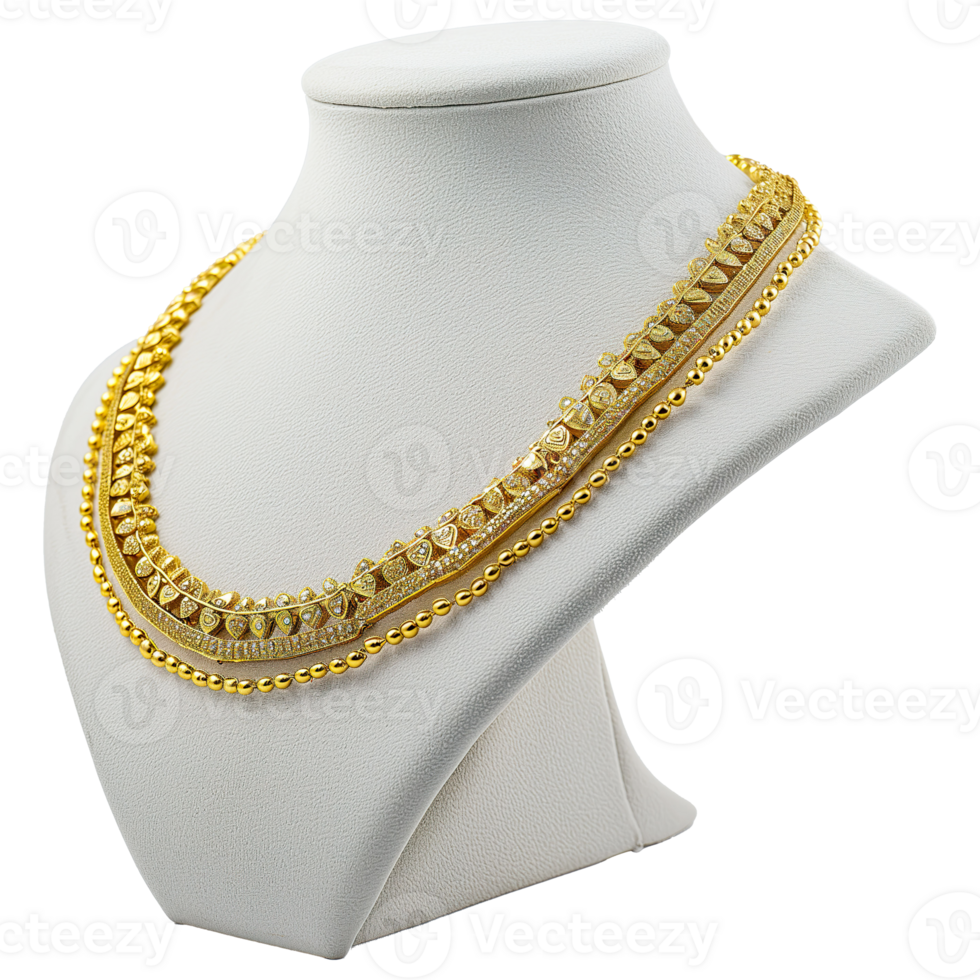This product image, likely a stock photograph, features two layered gold necklaces elegantly displayed on a white mannequin neck that mimics human shoulders. The first necklace consists of simple gold beads, exuding a timeless and classic look. In contrast, the second, more prominent necklace is adorned with a thick strand resembling leaves and features a striking band embedded with diamonds. The overall presentation highlights the necklaces' intricate details and luxurious appeal, set against a plain white background for emphasis. The image bears a repeating watermark reading "Vecteezy," indicating its stock photo origin.